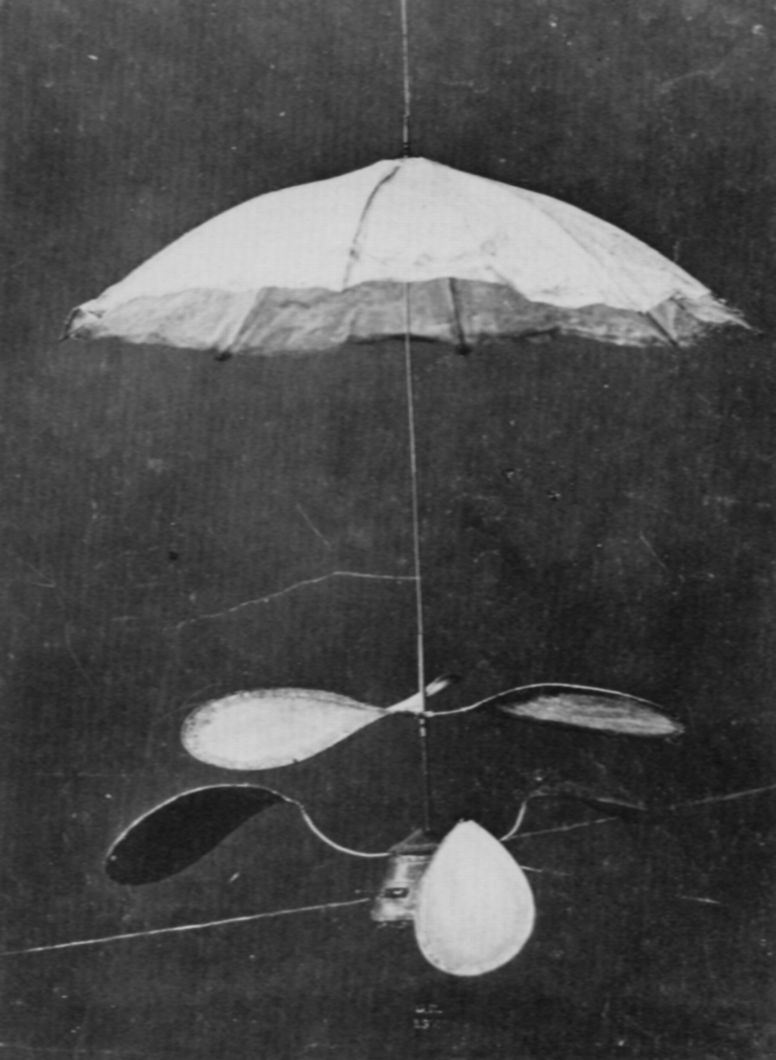The image appears to be an old, grainy black-and-white photograph, potentially dating back several decades, with no color. At the center is a white umbrella, extending vertically across the image. Unlike a typical umbrella, a thin pole stretches both above and below the canopy. Beneath the umbrella's top, multiple sets of metal objects resembling helicopter blades or rudders with rounded edges are attached to the central stem. The first set consists of two pieces while the lower set comprises three. These metallic elements are light in color, reflecting varying degrees of light, which creates a contrast against the dark, grainy, and somewhat torn background. The setup gives an impression of a peculiar device or an inventive art piece, possibly hinting at the concept of a "flying umbrella." No noticeable text is present in the image, which is fairly well-lit despite its antiquated appearance. The background also features scattered strands or ropes, adding to the overall impression of a meticulously arranged yet enigmatic creation.